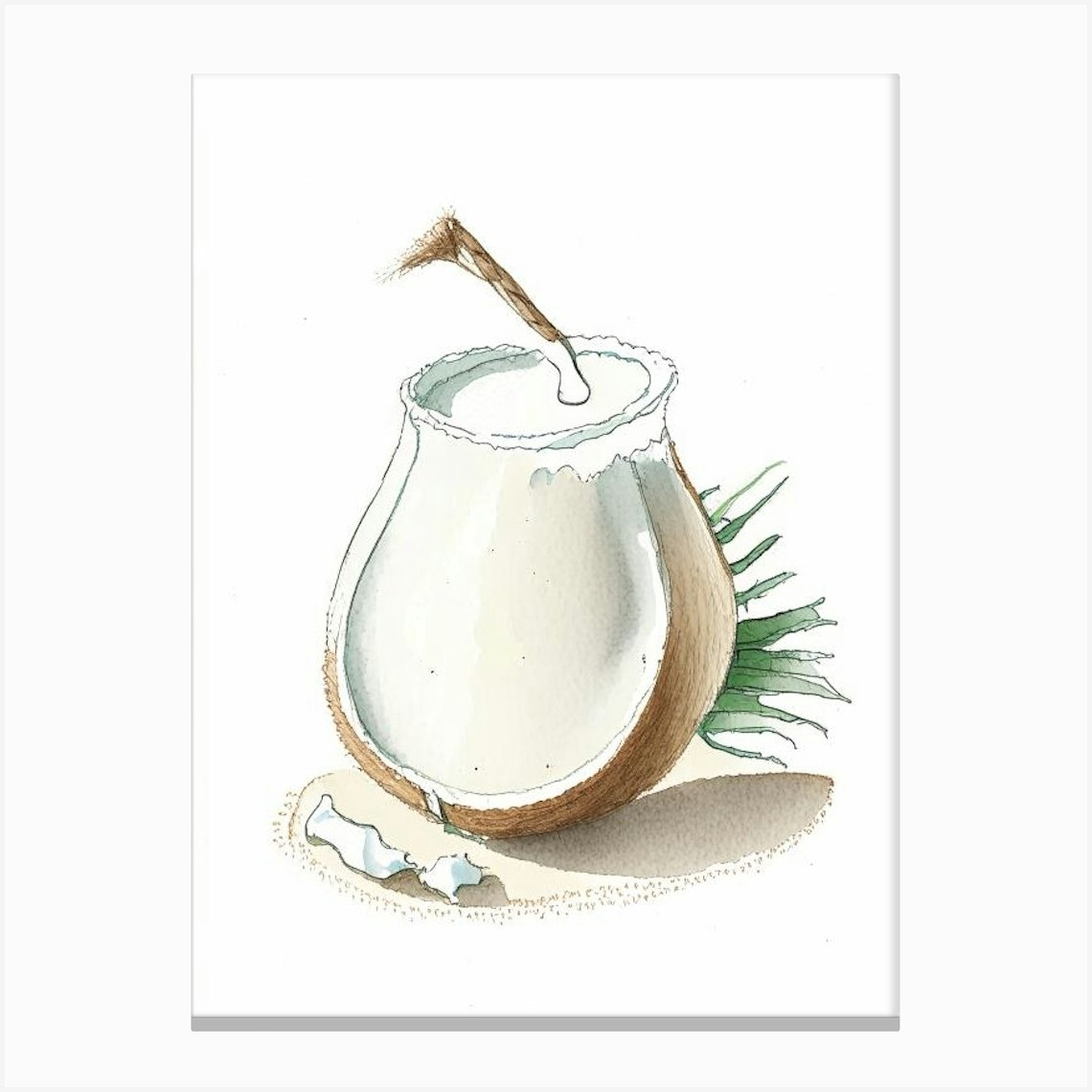The image is an illustration of a painting set against a white background, showcasing a central coconut that has been shaved and hollowed out to resemble a container, symbolizing coconut milk. This coconut has a brown outer shell and a meaty, white interior, which appears liquid in nature. The coconut, placed upright and central to the image, features a brown, slightly bent wooden straw inserted into it, adding a rustic touch. Behind the coconut, there are thin, green leaf-like structures, enhancing the tropical feel. To the right of the coconut, two white pieces of coconut flesh are placed, suggesting they have been broken off from the main shell. The coconut casts a shadow on the right side, indicating the light source is from the left. The setting and style of the painting focus on food, with an emphasis on the fresh, natural elements of the coconut.